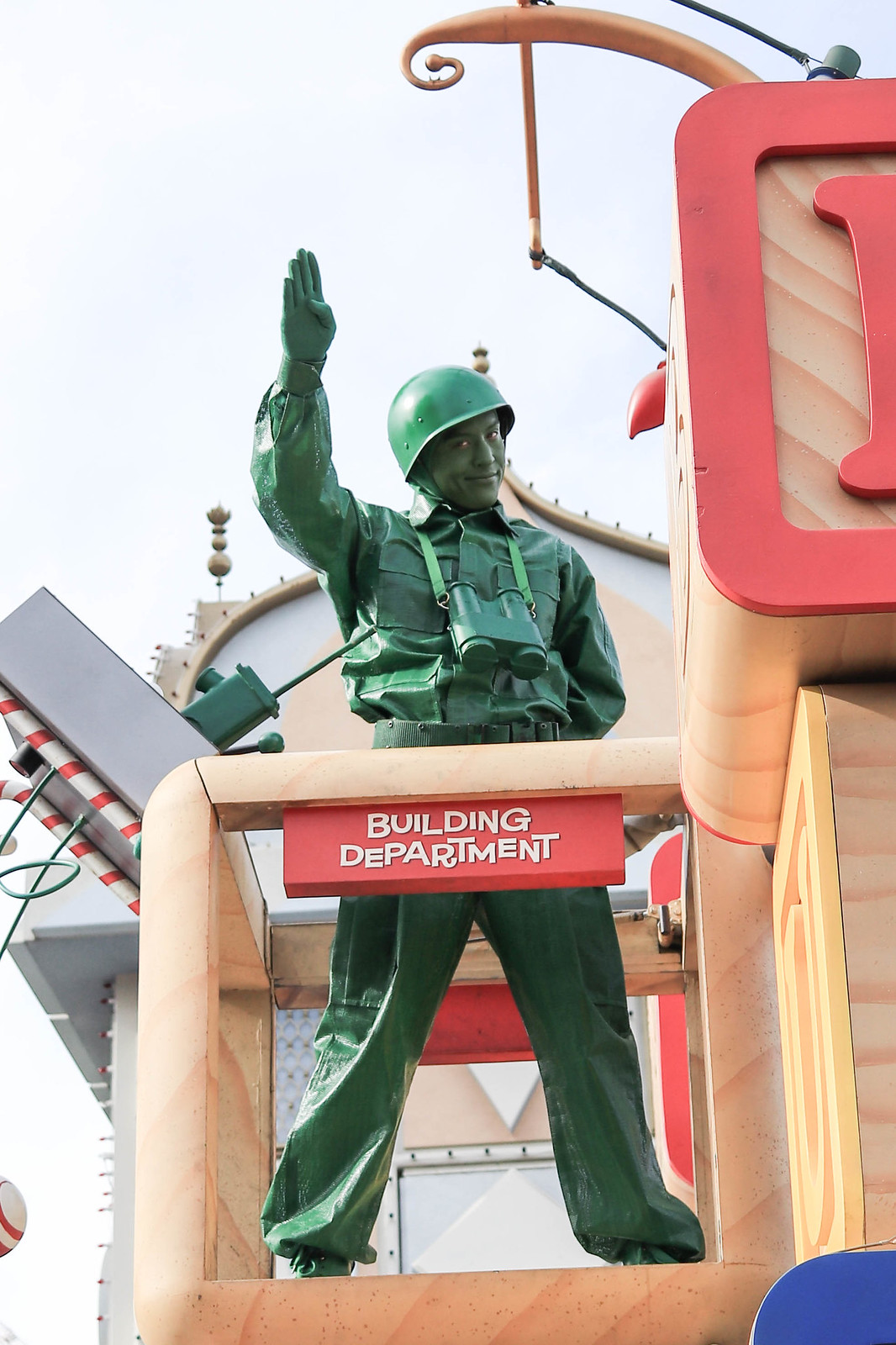This photograph depicts a strikingly life-like statue of a green army soldier at a Disney parade, possibly in Anaheim Disneyland Resort. The entire figure, from his face to his uniform—including a hard shell helmet, button-down collared shirt, binoculars, pants, and even his skin—is painted a uniform shade of green, lending him an almost toy-like appearance reminiscent of a character from Toy Story. The soldier's right arm is raised in a salute, with his head tilted slightly to the left while his eyes glance back towards the observer with a subtle smirk. The soldier stands on a structured platform adorned with multicolored blocks. Notably, a sign in front of him reads "Building Department" in all-capital white letters against a red background. Beside him, large candy canes and rows of chaser lights further contribute to the festive atmosphere, indicative of a parade float designed with meticulous attention to detail.